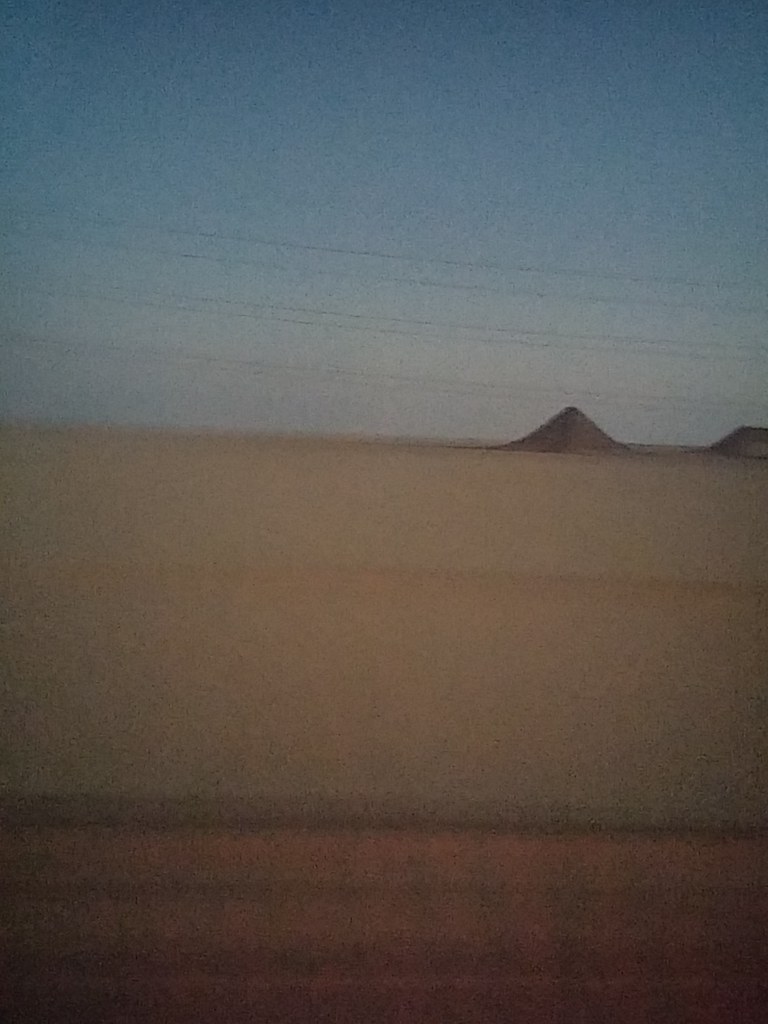This painting, with an upright rectangular orientation, depicts a serene outdoor scene. The upper portion, taking up nearly half of the canvas, showcases a gradient blue sky that transitions from a deep blue at the top to a lighter blue near the horizon. Near the horizon, pairs of thin black lines stretch horizontally across the canvas, reminiscent of power lines. Just above the midpoint, where the sky meets the earth, the palette shifts to a solid brown hue, representing the ground. On the right side of the painting, two small hills rise from the landscape, adding to the earthy texture. The brown ground gradually lightens as it descends, with the very bottom taking on a subtle orange-brown tint. Dark brown lines delineate the borders of the painting, adding a defined edge to this tranquil, rustic scene.